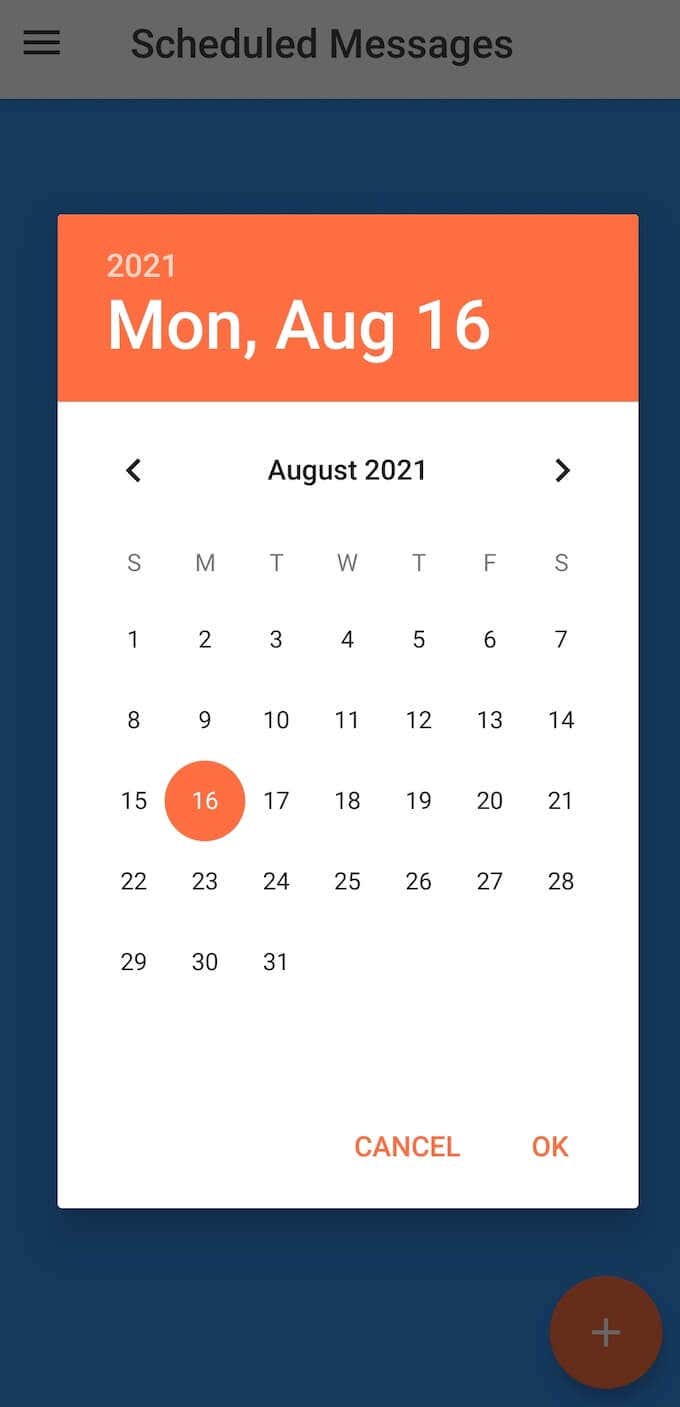This screenshot from a smartphone displays the "Scheduled Messages" screen, indicated by a dark gray header at the top. The main background of the screen is a navy blue color. In the foreground, there's a prominent date box that reads "2021, Monday, August 16th" in white text, with the month of August 2021 shown in a calendar format below.

Navigational arrows flank either side of the date box, allowing the user to move backward to previous months or forward to future months for scheduling purposes. Within the calendar, the date August 16th is highlighted in orange, signifying the current selected date.

Beneath the calendar, there are two options— "Cancel" and "Okay" — likely for confirming or canceling an appointment or message schedule. Additionally, there is a conspicuous orange box at the bottom featuring a plus sign (+), presumably for adding a new scheduled message or appointment.